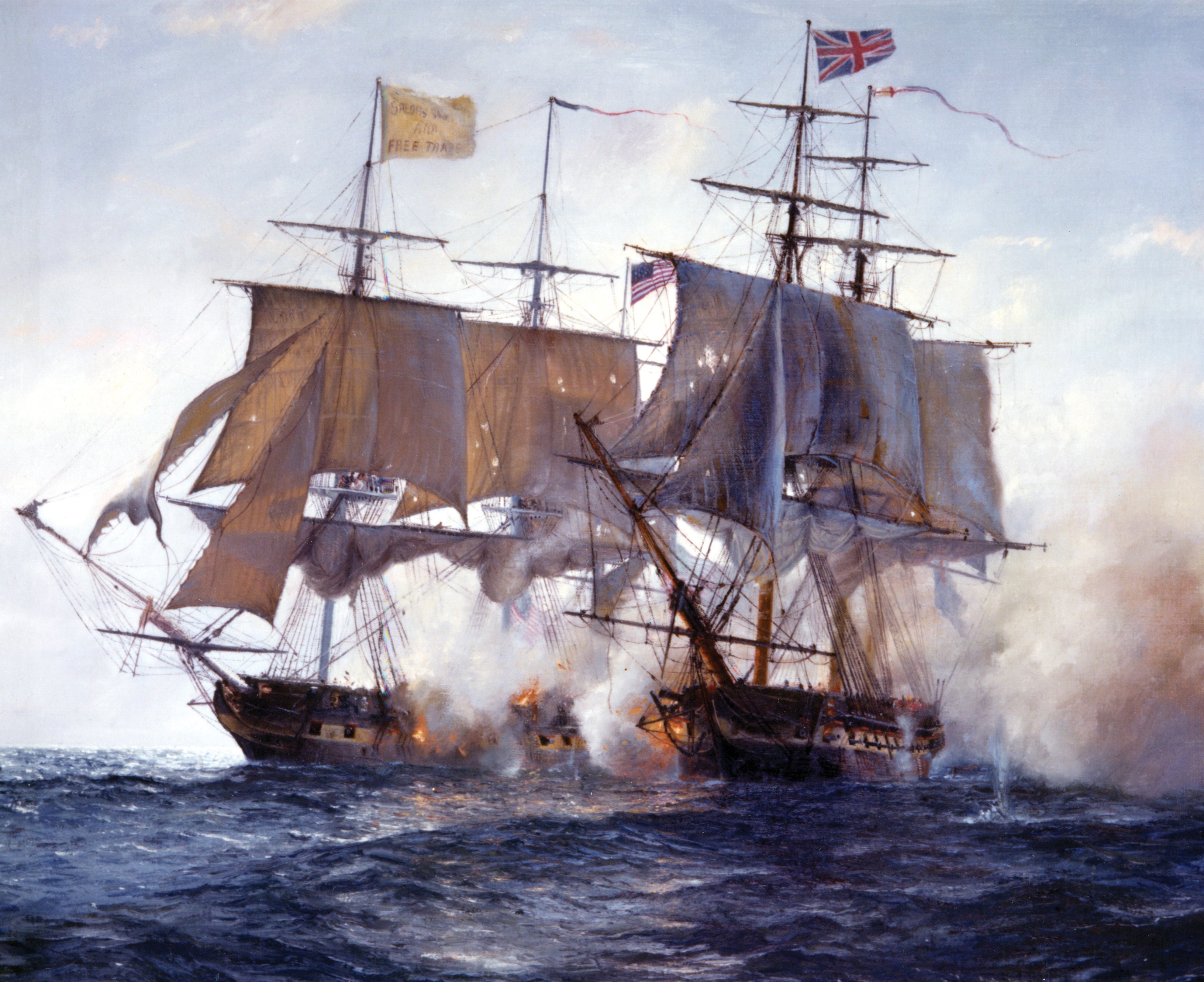This detailed oil painting or illustration showcases an intense naval battle between British and American ships, likely from two to three hundred years ago. The focal point is on two large sailboats exchanging cannon fire at close range, resulting in visible flames and thick plumes of smoke. The ship on the left flies a beige flag inscribed with the partially readable word "free," suggesting it may represent the American side. The British ship, identifiable by its flag, is positioned on the right. Both vessels are heavily engaged, with the American ship seemingly taking more damage, as evidenced by the more substantial smoke and fire emanating from it.

The ocean beneath them is dark blue and animated with splashes of white mist, contributing to the chaotic scene. The towering sails of both ships are predominantly beige but appear shadowed and weathered. There's also a third ship in the middle, caught in the crossfire and suffering substantial damage from both sides, adding to the drama.

The sky above is mostly clear with a subtle haze of clouds and mist, illuminated by a bright blue backdrop suggesting a sunny day, contrasting with the fierce battle below. The overall aesthetic with brownish, dark-toned ships and churning sea conveys a vivid and dramatic historical maritime conflict.